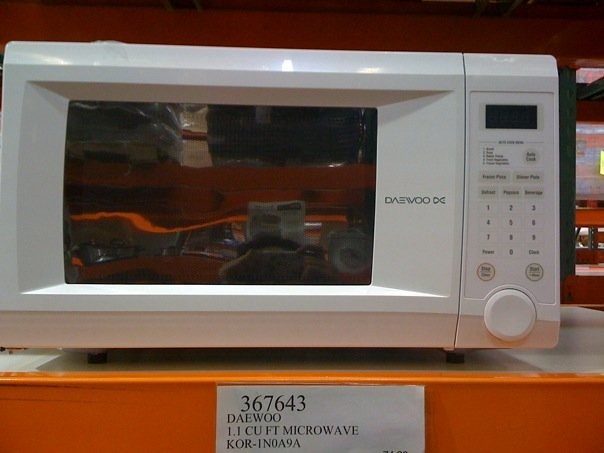This image depicts a white Daewoo 1.1 cubic foot microwave on the bottom shelf of a store display. The microwave features a black reflective window and a digital display, along with a dial on the right side which likely serves to open the door. A small, white sign with black font is attached below the microwave, displaying the item code "367643," the model "KOR-1N0A9A," and briefly mentioning the brand and capacity details. The shelf surface is white with a bright orange edge, and in the background, similar orange shelving units can be seen.